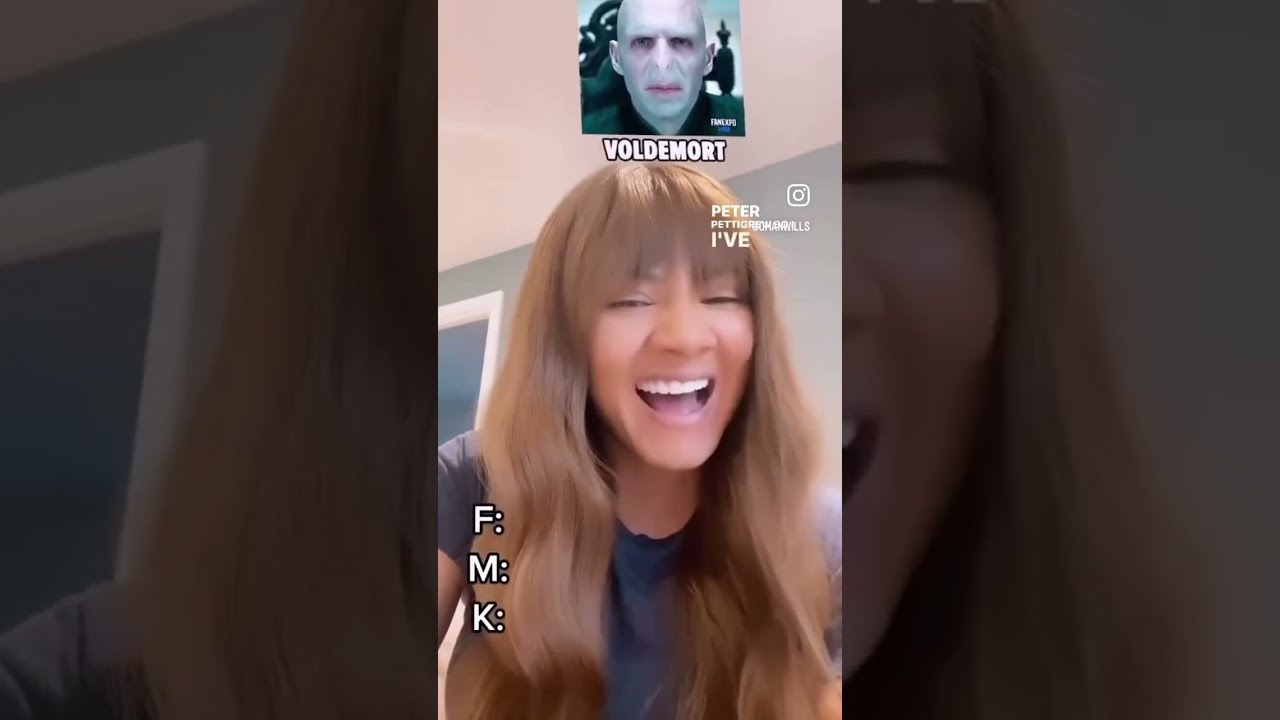This image appears to be a still from an Instagram live stream featuring a young woman with long brown hair and a blue or dark navy t-shirt. She is laughing while looking at the camera. Above her head is an inset photograph of Voldemort from Harry Potter, with "Voldemort" written underneath in all caps. To the right of this inset photo lies an Instagram icon with the word "LIVE" and some other text that includes the name "Peter." Overlaying the bottom of the image are the letters “F:M:K,” which suggests a "Fuck, Marry, Kill" game, possibly involving the character Voldemort. The overall aesthetic is that of a video freeze-frame typical of social media content.